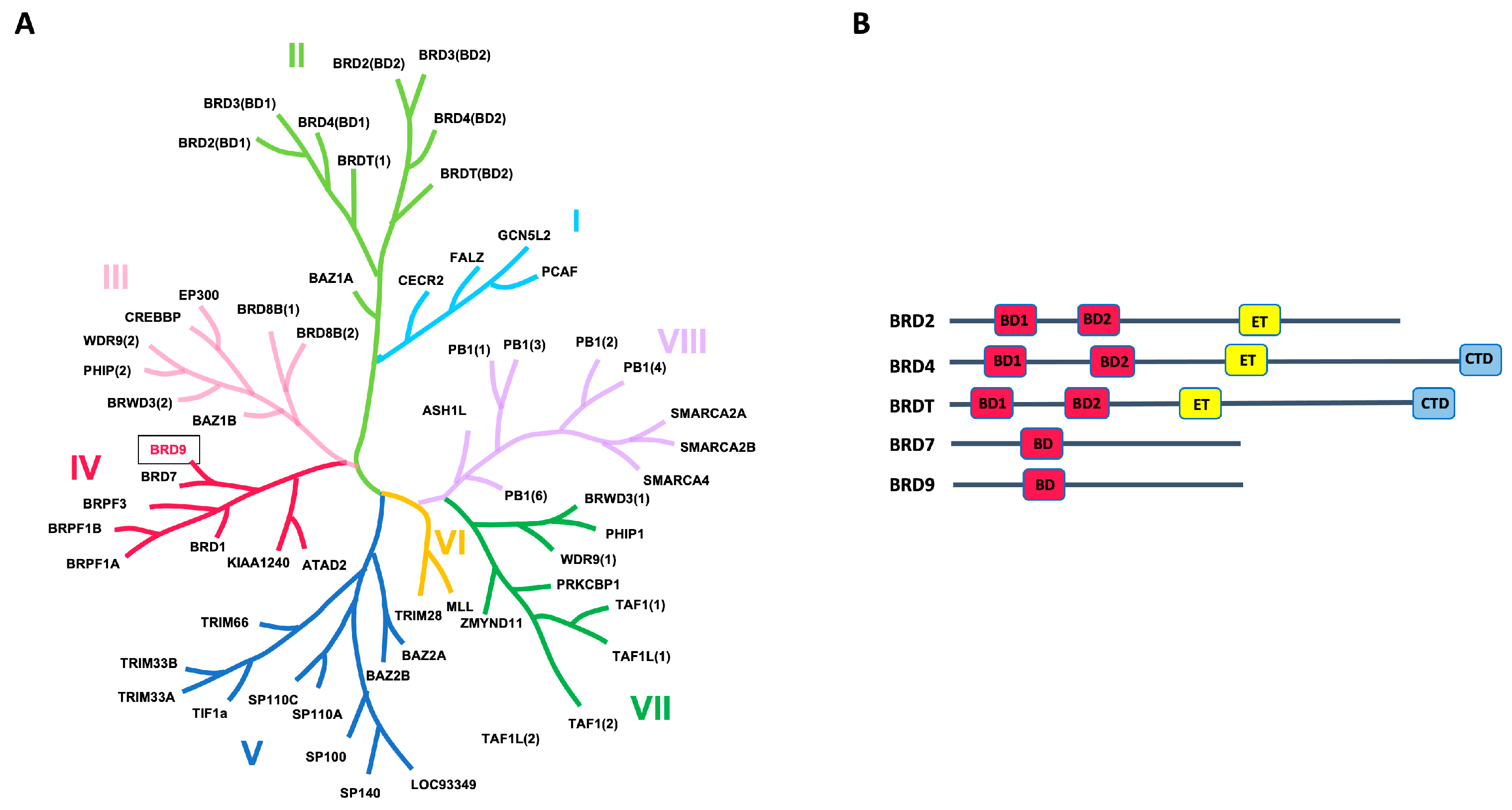The image is a detailed and colorful diagram resembling a branching tree or network of nerve endings, with various letters and abbreviations attached to the branches. The structure is organized with multicolored segments, which include green at the top, transitioning to pink, red, blue, yellow, and purple colors as it branches out. Each branch is labeled with identifiers such as BRD, BRD2BD1, and BRWD, specifying different chemical or biological entities. The branches are numbered in a counterclockwise fashion from 1 to 8.

To the right, there are five horizontal sliding scales, each beginning with the letters BRD, followed by a number. These rows include various squares—red, yellow, and blue—labeled with abbreviations like BD1, BD02, ET, and CTD. The scales appear to move horizontally across the screen, providing a detailed breakdown of different components associated with each BRD label. Additionally, on the left side of the image, labeled as part 'A', the branching pattern appears more vertical, underscoring its treelike appearance. The right section, marked as part 'B', houses the sliding scales and detailed annotations, creating a comprehensive visual that integrates both structural and categorical information on the subjects.